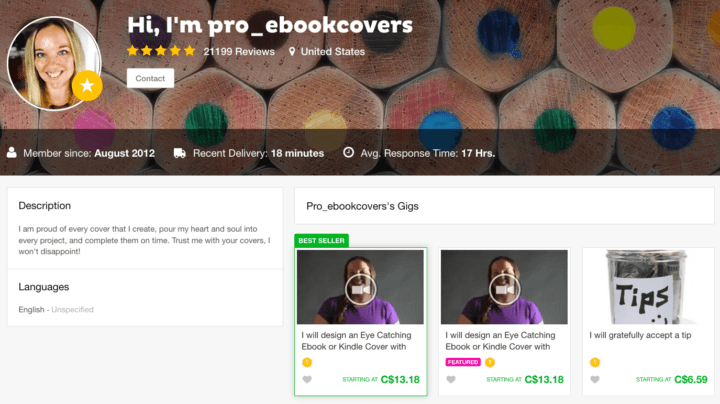The image showcases a profile on a freelance job platform where users can hire individuals for short-term gig work. The featured freelancer's username is "pro_ebook_covers," signifying her specialization in designing ebook covers. Her profile includes a profile picture adjacent to a yellow star icon. The top section of the webpage displays a vibrant background featuring the cut ends of colored pencils, revealing their colorful leads and the wooden parts, symbolizing creativity and artistry.

Her profile indicates that she has been a member since August 2012. Notably, her most recent delivery was made just 18 minutes ago, and her average response time is 17 hours. The freelancer's bio expresses her dedication and passion for creating ebook covers, stating: "I am very proud of every cover that I create. I pour my heart and soul into every project and complete them on time. Trust me with your covers; I won't disappoint." She communicates primarily in English.

Potential clients can hire her by clicking on various purchasing options available on her profile, one of which reads, "I will design an eye-catching ebook or Kindle cover." Additionally, there is a section where clients can leave tips for her services.